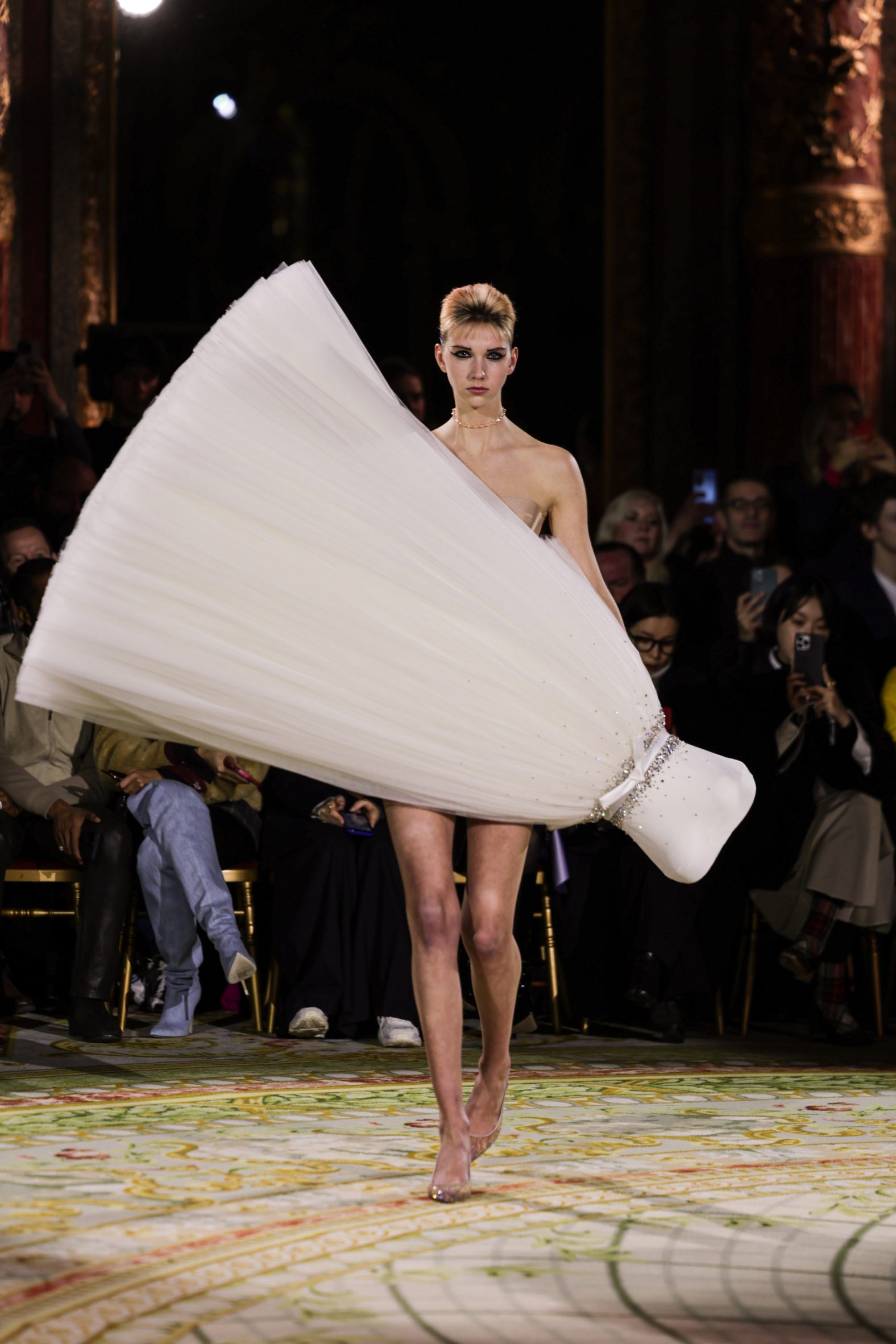A high fashion model with short blonde hair is captured walking down a runway, wearing a unique, avant-garde dress that appears rotated and diagonally draped across her body. Her legs and the upper portion of her chest are visible, with a hint of a nude halter near her left shoulder. The dress is adorned with glitter around the waist and features a central bow. She wears high heels and completes her look with a necklace, red lips, and dark eye shadow. The audience behind her, some holding up phones to capture the moment while others watch intently, suggests a vibrant fashion show setting. The ground beneath the model is decorated with abstract shapes and lines in green, red, orange, beige, and yellow, while the overall background remains dark, emphasizing the model's striking presence on the runway.